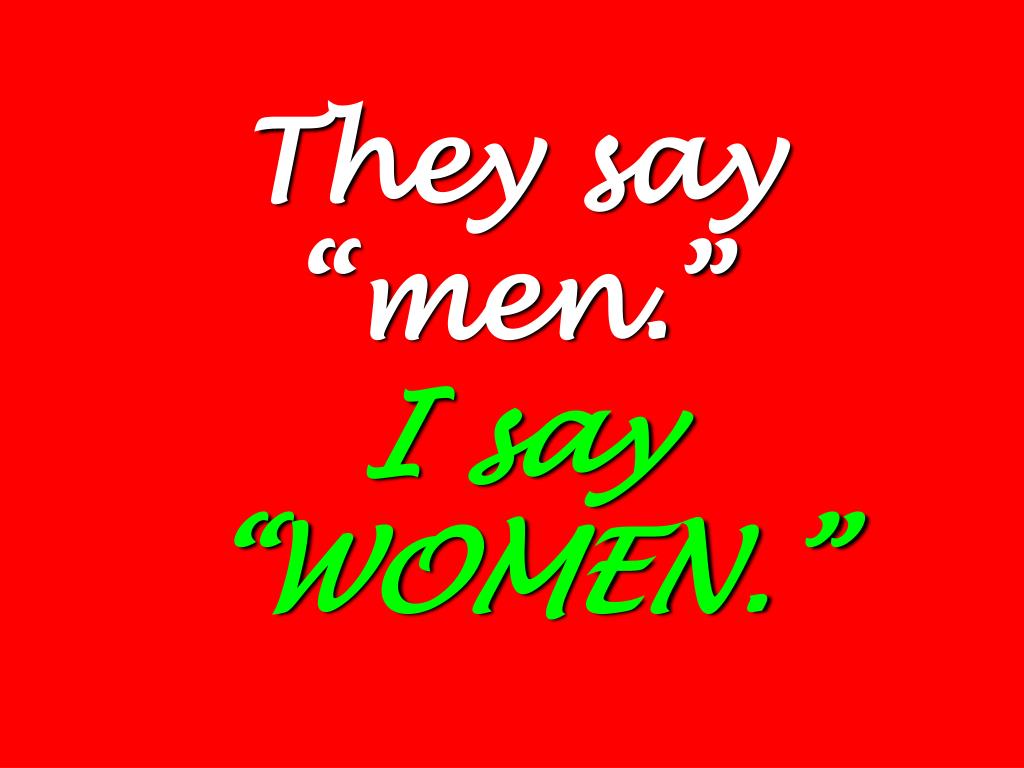The image features a square or rectangular design with a dark red or orange background. At the top, in bold white cursive, is the phrase "They say," followed by the word "men" in parentheses and printed in white. Below this, in bright green cursive, is the phrase "I say," followed by the word "WOMEN" in all capitalized letters and also in parentheses. The overall impression is a feminist statement highlighting the contrast in addressing humanity by emphasizing "women" instead of "men." The clear and uncluttered layout draws immediate attention to the contrasting colors and the impactful message.